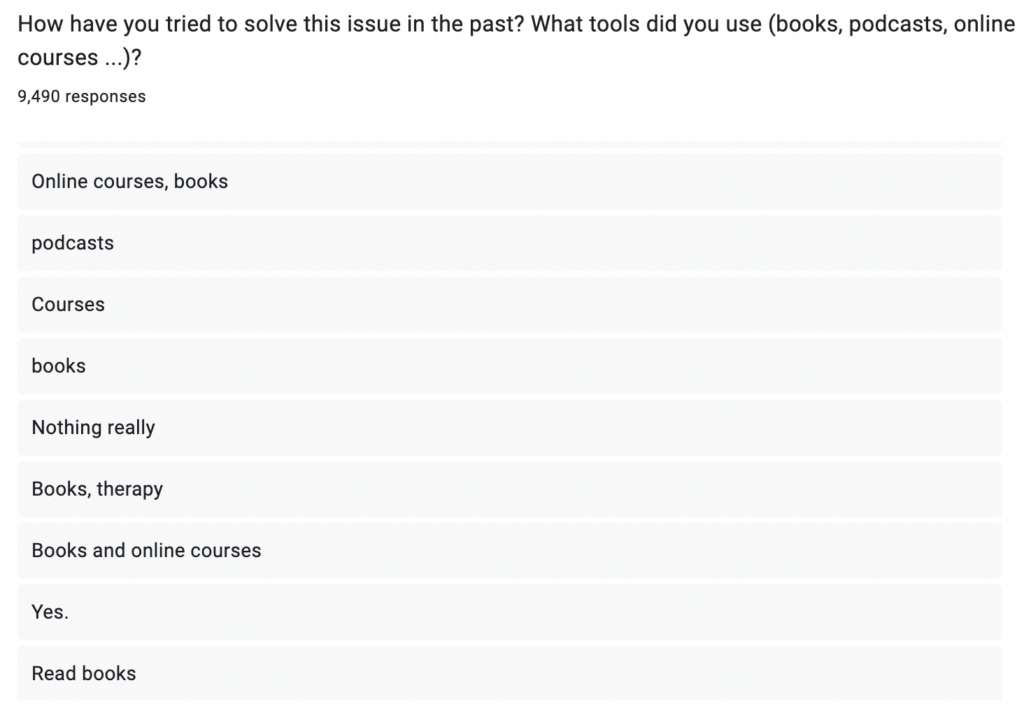The image displays a detailed question from a dialogue box in bold text: "How have you tried to solve this issue in the past? What tools did you use? Books, podcasts, online courses, etc." The question garnered a total of 9,490 responses. Below the question, various options are listed for respondents to select as tools they have previously used to tackle the issue. The options include:

1. Online courses
2. Books
3. Podcasts
4. Courses
5. Nothing really
6. Therapy
7. Books and online courses
8. Yes (implying a general affirmation)
9. Read books

These responses showcase a range of single and combined tools utilized in the past. The list appears to be part of a questionnaire aimed at gathering statistical information on the most common methods people employ to address certain issues. The responses reflect whether individuals prefer singular approaches, like reading books or listening to podcasts, or a combination of methods, such as using both books and online courses, thereby shedding light on diverse problem-solving strategies.